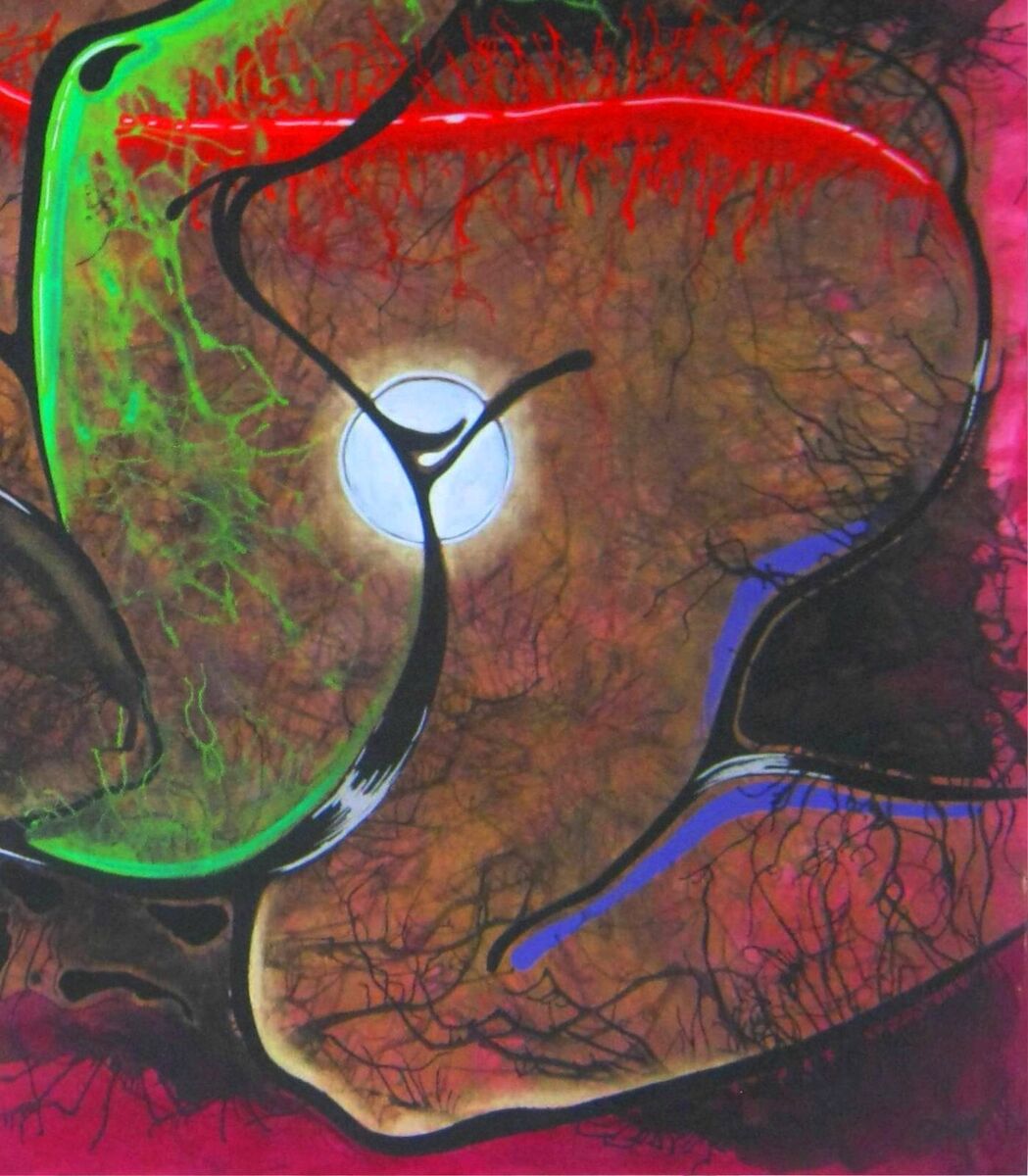This image showcases an intriguing and abstract piece of artwork on a rectangular canvas, where the height is half the length of the width. Dominated by a striking palette of red, black, white, and neon hues, the painting features various black curved lines interspersed with white highlights, adding texture and depth. These lines are complemented by finer black tendrils and vein-like structures that weave throughout the composition.

At the center of the artwork lies a prominent white circle bordered in black, which exudes a small, radiant yellow halo, giving the impression of a celestial body, possibly a sun or moon. The top left quadrant features vibrant, neon green tendrils, contrasting sharply with the predominantly darker colors. A distinct red line extends from the top left corner towards the top right, intersecting the green tendrils and adding a dynamic element to the scene.

The canvas also contains patches of blue and pink amidst the dominant reds, creating a highly eclectic and vibrant visual feast. The overall aesthetic is both abstract and slightly disorienting, with the chaotic mix of colors and lines evoking images of blood vessels or an anatomical landscape. Despite the low resolution and slightly blurry texture, the painting stands out for its bold use of colors and complex interplay of shapes and lines.